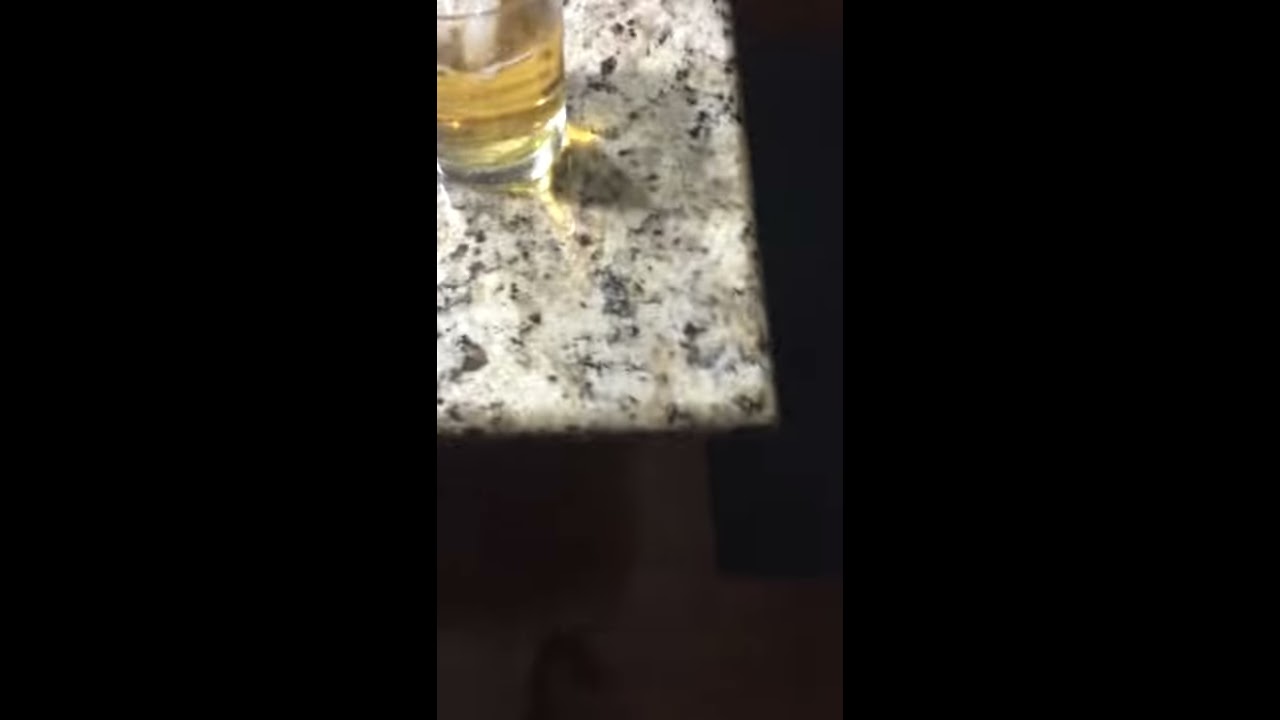The image is vertically oriented and divided into three sections, with the left and right thirds blacked out. The main focus, positioned in the center, depicts the corner of a table or countertop taken indoors. Despite the overall dark ambiance, fine details emerge from the low-resolution, slightly blurry shot. The table or countertop displays a faux marble surface, a light base color interlaced with speckles of black and brown, evoking a marbling effect. Occupying the upper left corner of the table is the lower portion of a cylindrical glass bottle containing a light amber-colored liquid. The exact nature of the liquid is indistinct, resembling either apple juice or whiskey. The periphery below and to the right of the table is steeped in darkness, obscuring any potential details of the flooring or objects in those areas.